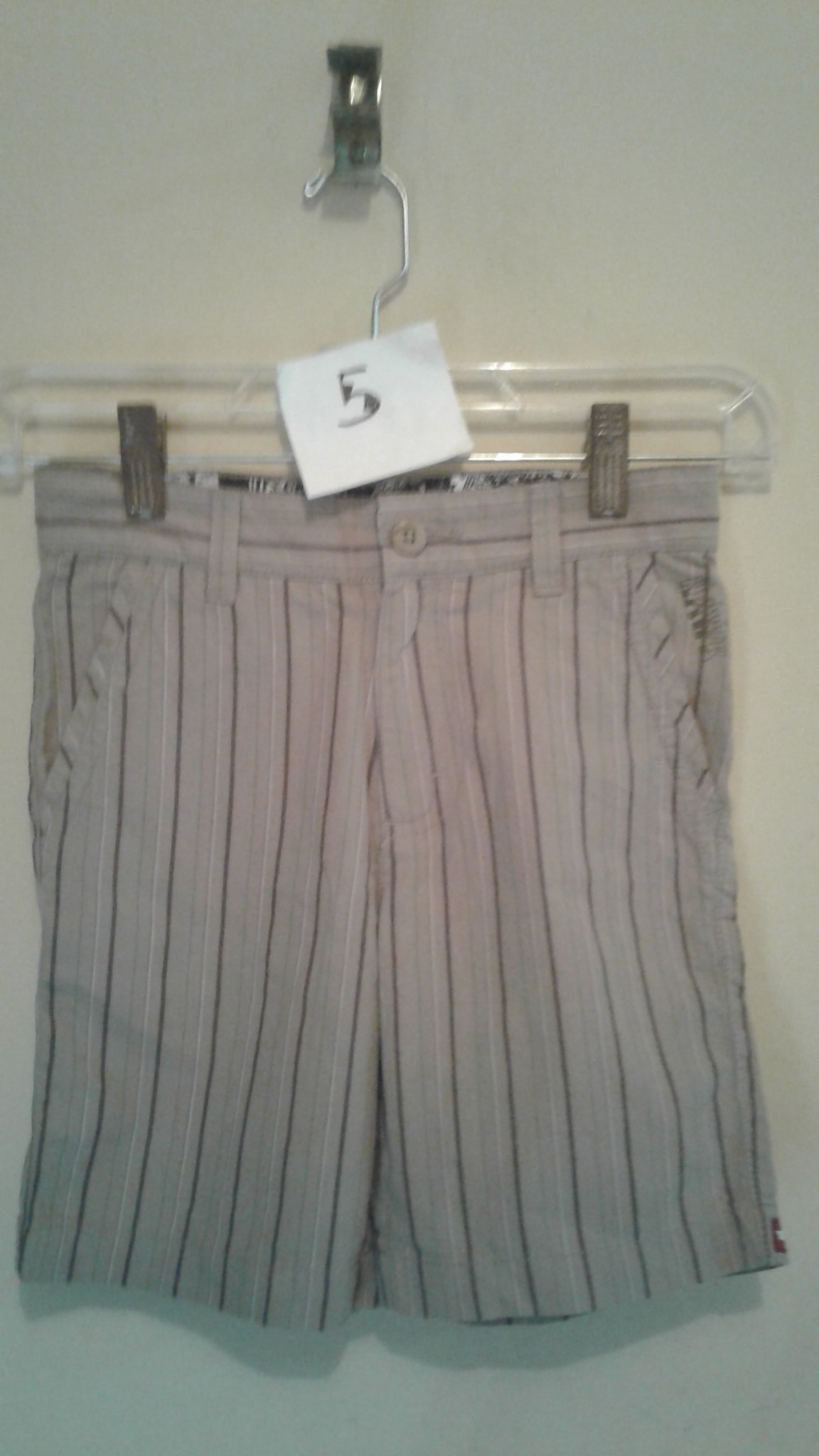This image captures a pair of gray, vertically striped shorts hanging on a transparent plastic clothes hanger, suspended from a silver metal hook on a white wall. The shorts feature thin pinstripes, alternating between dark and white, running vertically down their length. They are equipped with side pockets, visible belt loops, and a single button on the waistband. The hanger, commonly used in shopping outlets, includes dual clips securing the shorts and a white square piece of paper with the number 5 affixed to it. The white wall behind casts a subtle shadow of the shorts, enhancing the black-and-white feel of the image.